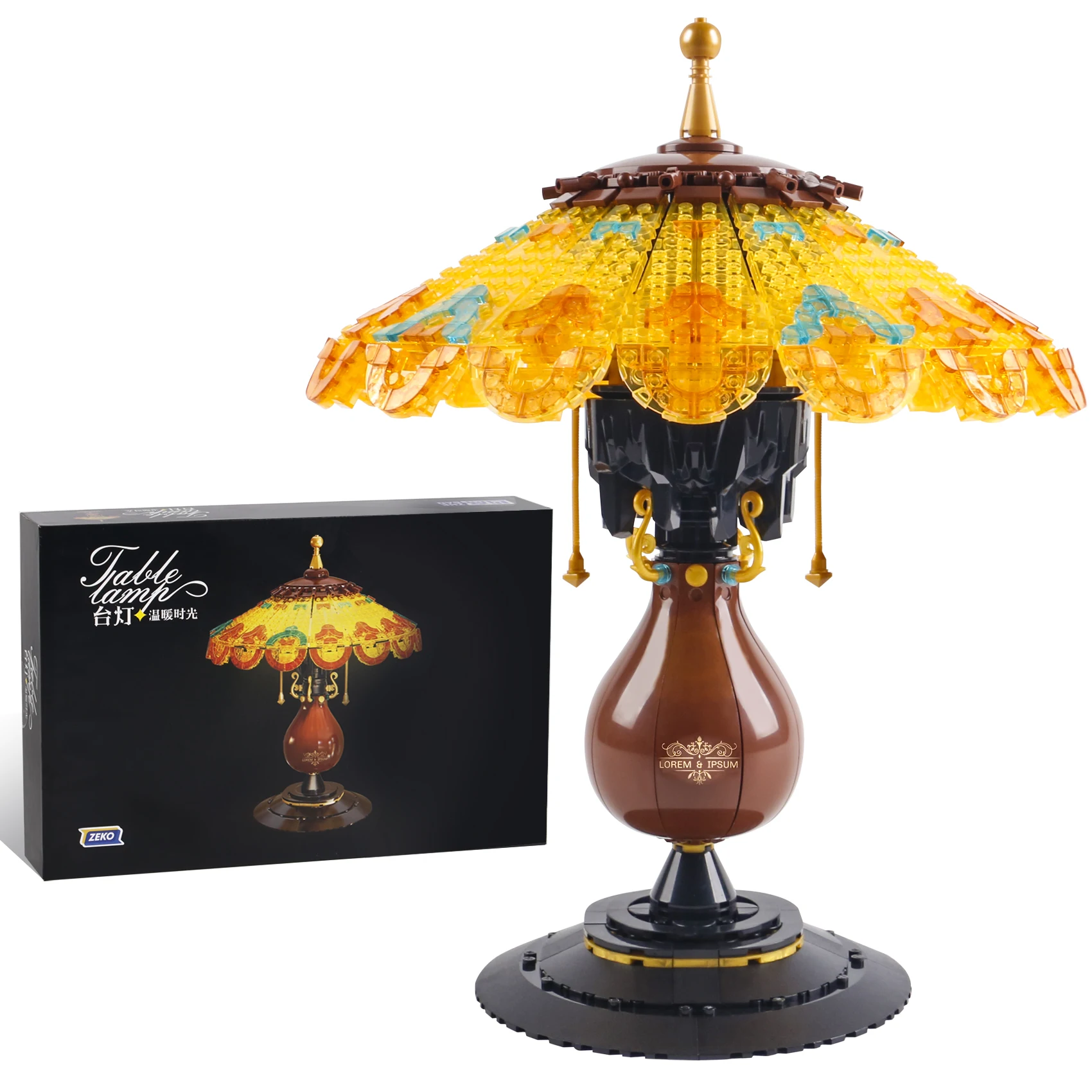The image depicts a small, intricately detailed lamp designed in a Lego style, situated with its packaging in the background. The lamp features a black circular plastic base supporting a vase-shaped, brown middle section etched with a gold "Lorem Ipsum" insignia. Above this section, two golden strings hang down, mimicking pull-cords for turning the lamp on and off. The lampshade, constructed from transparent yellow Lego pieces with blue accents, culminates in a brown top with a gold point. The packaging, positioned to the left, is a sleek black box displaying an image of the lamp on its front, with "Table Lamp" written in white lettering in the upper left corner, and some additional writing in an Asian script. This stylized lamp is both a functional piece and a decorative object, blending playful Lego elements with classic lamp design.